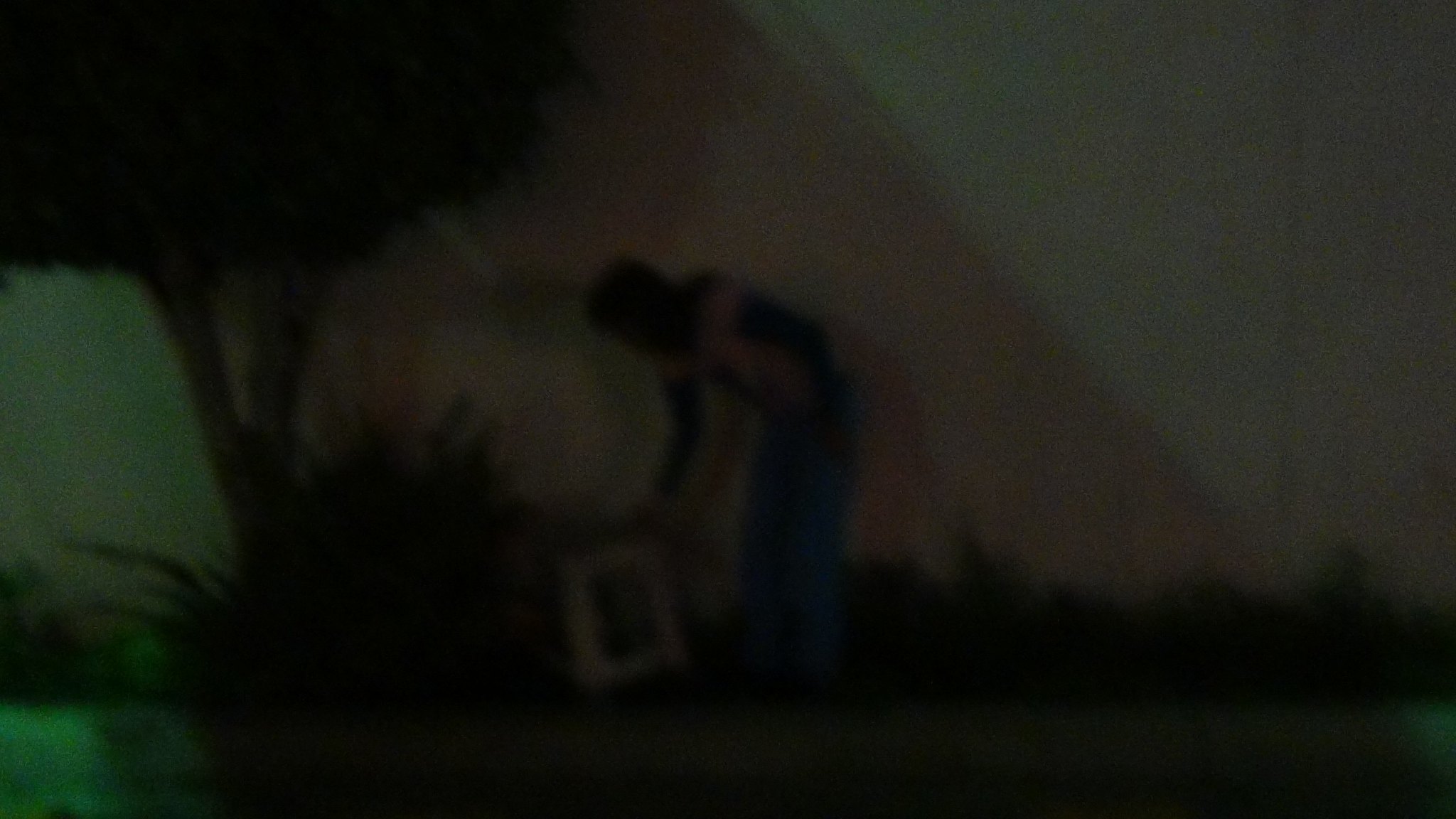In this artistic, blurred image resembling a painting, the left side contains a small body of water adjacent to a patch of grass. Directly behind this grassy area, a tree and a bush are prominently featured. A wall painted in varying hues of green and pink stands behind the foliage, serving as a colorful backdrop. The scene includes a dark-skinned gentleman dressed in jeans and a long-sleeved shirt, who appears to be placing a picture frame in front of the bush. The image also shows a continuous line of bushes extending across the entire frame, with a stretch of grass in the foreground. The purpose of positioning the picture frame in front of this bush, positioned before the tree, remains unclear.